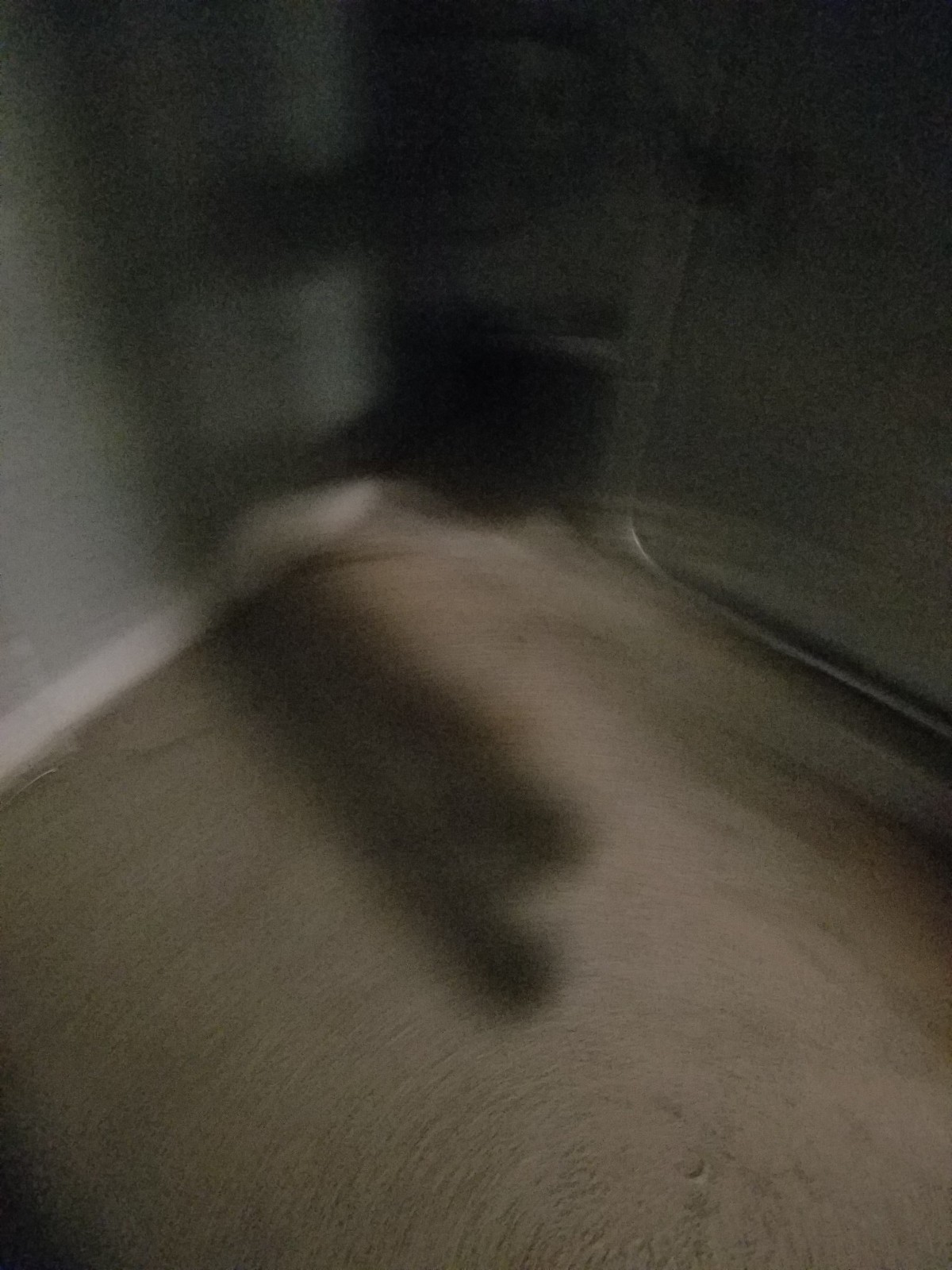The image depicts a vertically shot, blurry interior scene, possibly of a small, cramped room or closet. The room features light tan carpeting and gray-painted walls with white trim along the bottom edge. The photo captures the corner where two walls meet, extending upwards from about halfway up the image to the top, with the corner itself creating a notable shadowy area. Along the right side, there's a partially visible silver metallic frame, likely the bottom half of a clothes rack. In the center, obscured by shadows, there appears to be a built-in white bookshelf or a doorway opening with white trim. The left wall is described as having a greenish hue with two distinct shadows stretching from the floor to the top of the wall. Dominating the foreground are several tall, rectangular shadowy protrusions. The overall mood is dark, with the shadows contributing to a sense of depth and mystery. It remains unclear whether the image is an actual photograph or a drawing with heavy brushstrokes creating the blurred and shadowy effects.